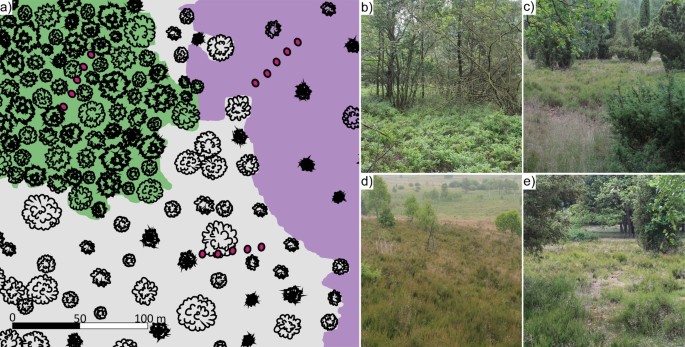The image is a rectangular collage split into two main sections. On the left side, labeled "A," is a detailed, hand-drawn aerial map of a field, featuring various colored sections and labeled areas. The map highlights different zones: a dense forest area depicted in green and black, a more sparsely treed region in white, and another portion marked with purple, filled with dark purple dots. Additionally, a distance key is visible at the bottom left of this map.

On the right side are four distinct photographs labeled "B," "C," "D," and "E," arranged in a two-by-two grid. These photos capture different ground-level views of the field and forest area illustrated in the drawing. The images predominantly feature green grass, trees, and bushes, giving a vivid representation of the natural landscape depicted in the map. The overall color scheme of the collage is dominated by green, white, and purple tones, effectively merging the artistic aerial perspective with the realistic ground-level photographs.